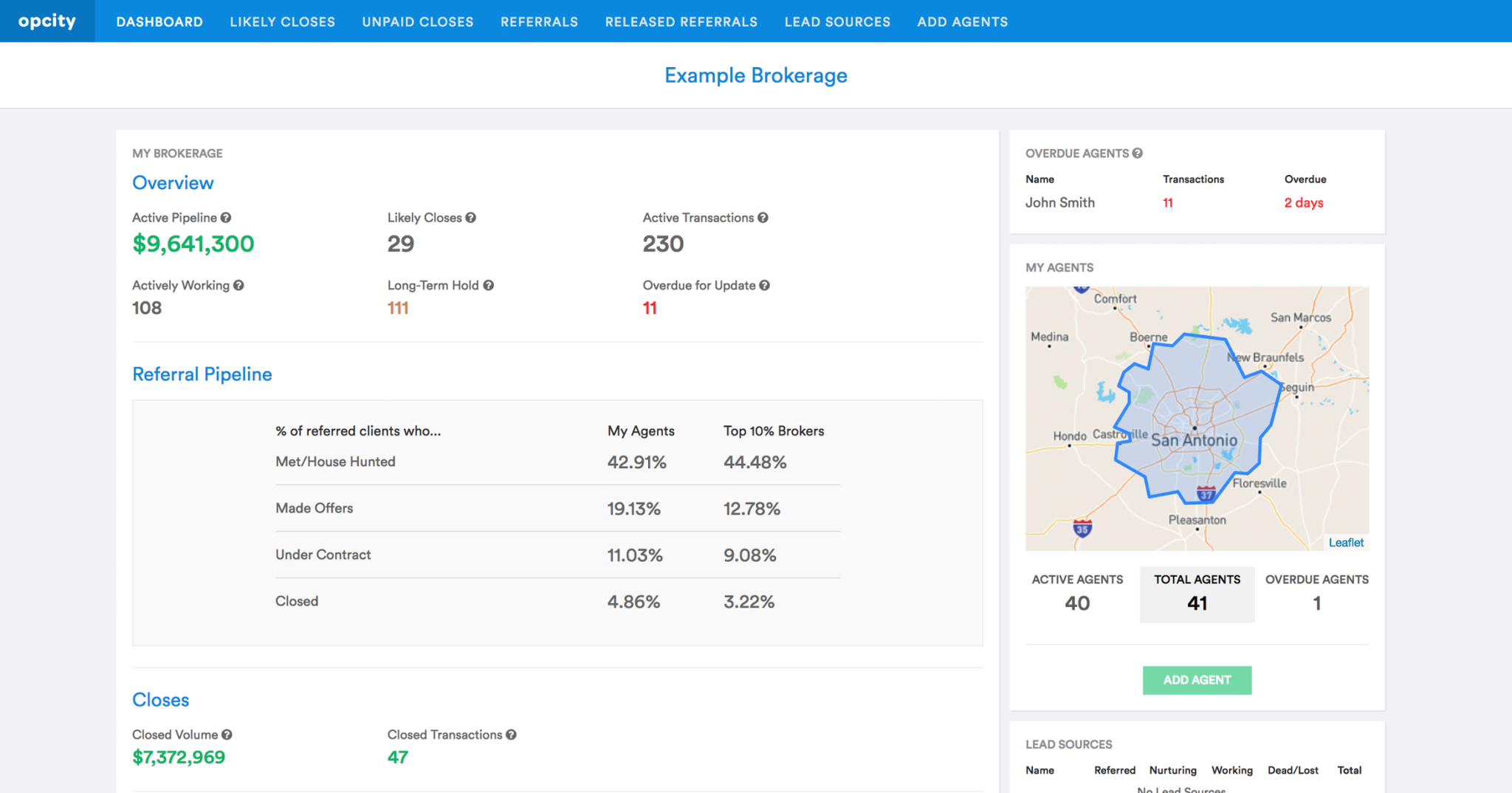Here is a cleaned-up and detailed caption for the given image:

---

Screenshot of the Example Brokerage dashboard interface featuring a top blue menu bar with white text options: Op City, Dashboard, Likely Closes, Unpaid Closes, Referrals, Released Referrals, Lead Sources, and Add Agents. The interface is divided into two primary columns, with the left column being more expansive. 

The left column is titled "My Brokerage Overview" and displays an "Active Pipeline" valuation of $9,641,300 in green text against a white background. This section also includes various other text and numbers, some highlighted in red and black, indicating different data points. 

Additionally, there is a "Referral Pipeline" section accompanied by a chart, and a "Closes" section featuring more figures marked in green.

On the right-hand side of the page, there's a segment named "Overdue Agents," and below it a "My Agents" section. This column also includes a detailed map of San Antonio with the San Antonio area highlighted in blue.

---